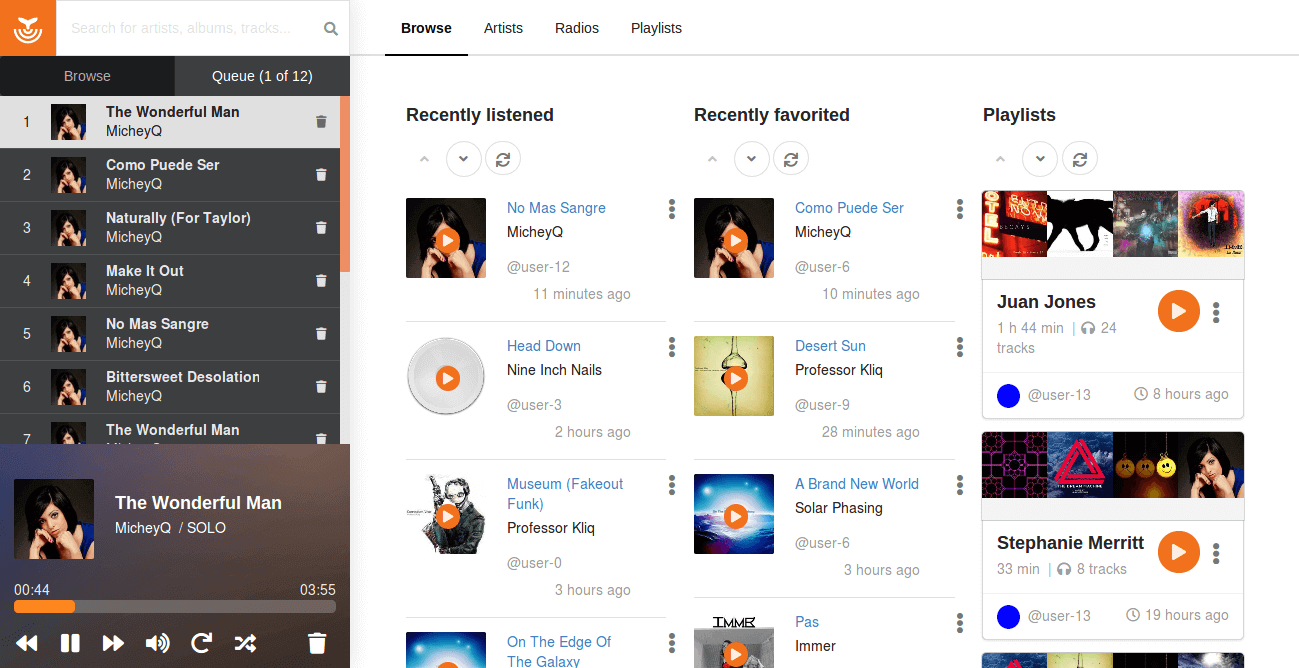The screenshot displays a music streaming application's interface, highlighting several features and recently interacted content. At the top of the screen, there are options for "Browse Artist Radio Playlist" alongside sections for "Recently Played," "Recently Favorited," and "Playlist."

In the "Recently Played" section, the entries include:
- "No Mas Sangre" by Miki Q, played 11 minutes ago.
- "Head Down" by Nine Inch Nails, played two hours ago.
- "Museum" by Fake Out Funk, Professor Click, played three hours ago.

In the "Recently Favorited" section, the highlighted tracks are:
- "Como Puedo Ser" favorited 10 minutes ago.
- "Desert Sun" by Professor Click, favorited 10 minutes ago.
- "A Brand New World" by Solar Phasing, favorited three hours ago.
- "Pause" by Immer.

The "Playlist" section shows:
- "Juan Jones," with a total playtime of one hour and 44 minutes, marked with an orange play button.
- "Stephanie Merritt," with the play button, last played 19 hours ago.

On the left sidebar, the options to either "View" or "Browse" playlists are visible, finalizing the display as a comprehensive overview of the user's recent activity in the music streaming app.